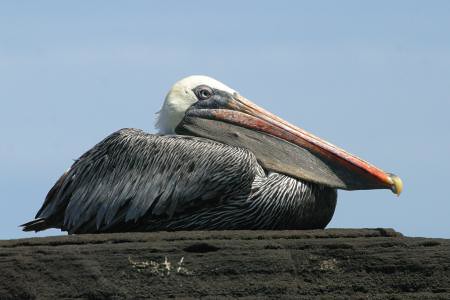In this outdoor, daytime photograph of nature, a large seagull, possibly mistaken for a pelican due to its size and beak, is sitting on a gray rock or potentially a piece of driftwood or wooden post, directly in the center of the image. The bird's feathers display a mix of black, white, and gray, with its white head contrasting against the bright blue sky. The seagull's beak is predominantly dirty orange with a hint of pink and white at the tip, resembling an extra small beak. Its wings are folded neatly at its side as it looks to the right of the frame. The clear, blue sky, occasionally interrupted by a few sparse clouds, provides a serene backdrop for this natural scene. The vibrant colors in the image include the blue of the sky, the gray of the rock or wood, and the multi-hued feathers and beak of the bird. No text is present in the image, fully immersing the viewer in the tranquil, daylight setting.